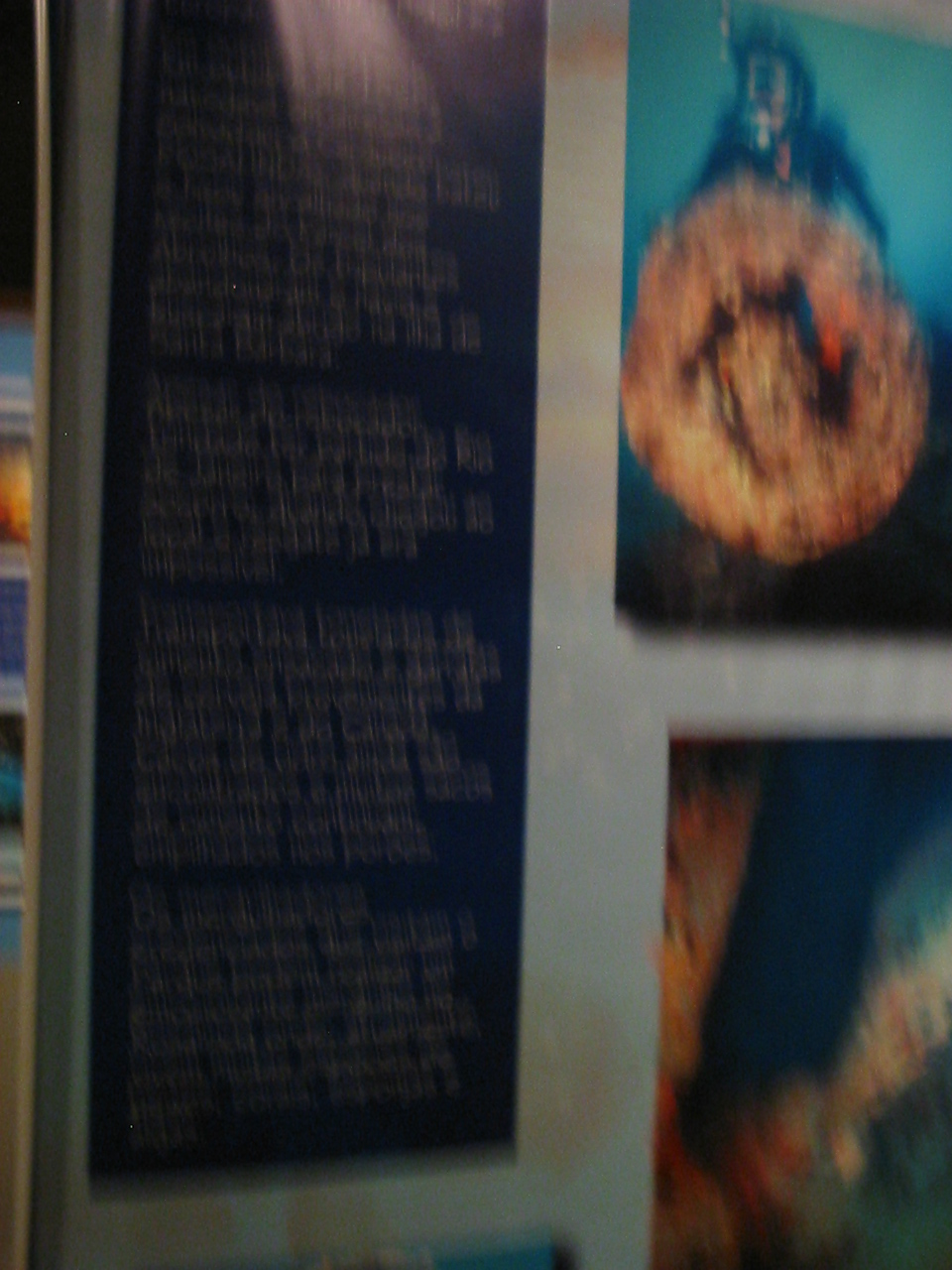This is a super blurry photograph of a magazine page, printed on glossy paper. The image is in portrait orientation. On the left side of the page, there is a tall, dark, almost navy blue rectangular box filled with dense, light peach or light-colored text, which is too blurry to read or identify the language. On the right side, the page features two rectangular images. The upper image has an aqua background with a scuba diver holding a large, fiery bright orange ball-like object, which might be a heavily calcified and rusted structure or coral. In the lower section, there's the start of another underwater image, also featuring similar bright, fiery structures. The overall scene gives an impression of an underwater exploration or dive, with vibrant and eye-catching elements contrasted against the darker waters.